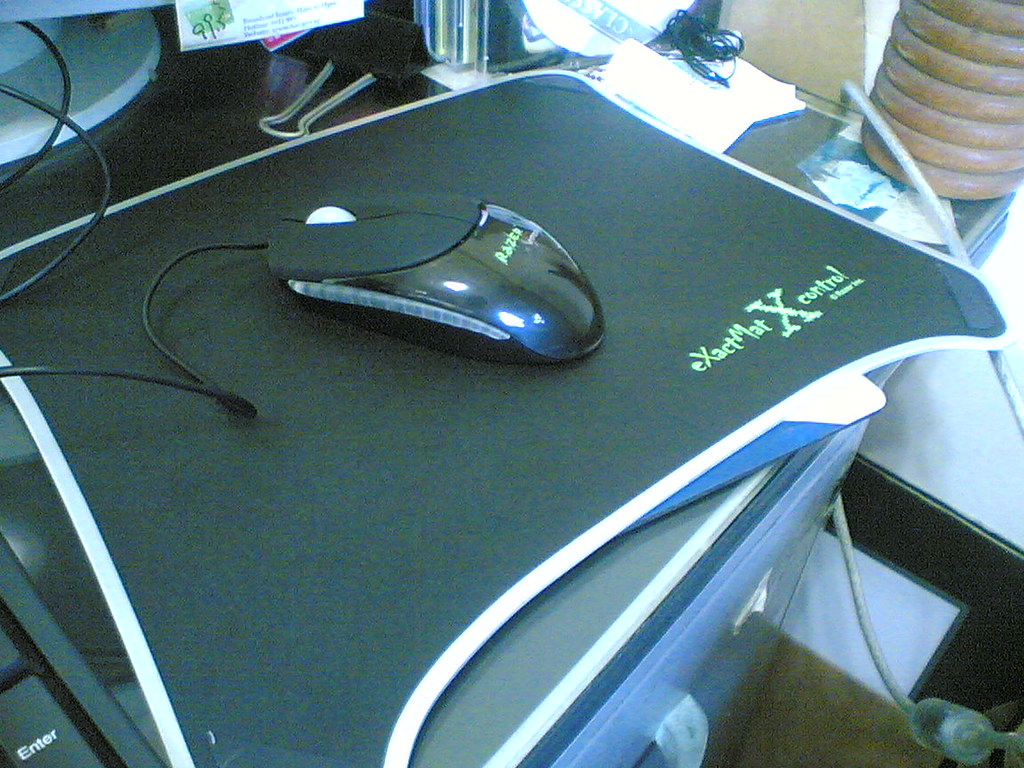In this color photograph, we see a detailed setup featuring a black mouse pad with a white bordered edge situated on a grey desk. The rectangular mouse pad, titled "EXACT MAT X CONTROL," is distinguished by its unique irregular corners at the bottom right and eerie green text. Centrally located on the pad is a black computer mouse branded "RAZER," which features a white mouse wheel, a grey line on the side, and glossy black accents that reflect the room's overhead lighting. A black wire extends from the mouse towards the left side of the photo, disappearing out of frame. Surrounding the mouse pad is a mix of clips, decorations, and miscellaneous clutter, adding context to the environment. In the top left corner of the image, part of a white computer monitor base is also visible. The overall quality of the image is somewhat fuzzy, but the composition clearly focuses on the mouse and mouse pad as the main subjects.